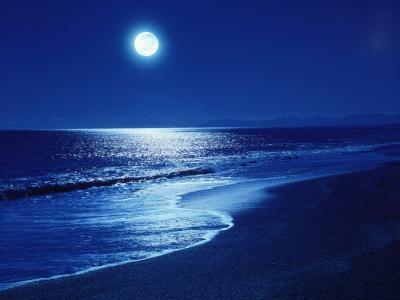The image portrays a serene nighttime beach scene dominated by shades of blue. The sky, a deep yet not entirely black hue, features a bright, glowing white moon slightly left of center, casting a tranquil ambiance. The moonlight reflects off the ocean, which appears in darker blue tones. Gentle waves lap onto the shore, creating a rhythmic pattern that conveys a sense of movement. Though the exact color of the sand is obscured by the darkness, it blends into the overall blue palette. In the horizon's distance, faint outlines of mountains are visible, adding depth to the scene. The photograph, captured in landscape mode, is vivid and highly detailed, emphasizing the glowing moon, the reflective water, and the tranquil, rippling waves of the ocean.